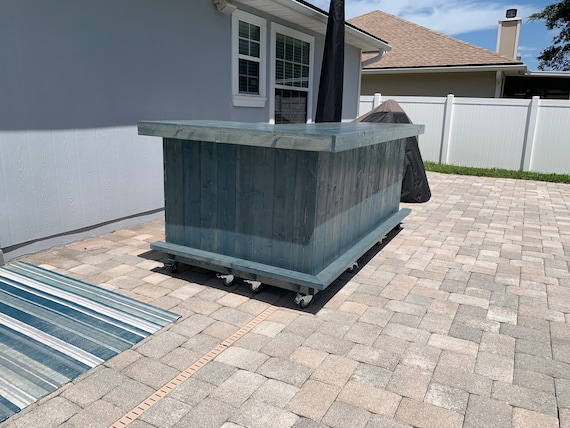The photograph captures a sunny day scene of a fenced-in back deck area of a house, with a blue sky adorned with white clouds. The main house, visible behind a white plastic fence, features a light brown, triangular roof with a chimney, and it has grey exterior walls with large doors and windows bordered in white. The stone patio deck is paved with square-shaped brick tiles. On the deck, there is a prominent, potentially mobile, high-quality hot tub-like structure on wheels, painted in blue and grey. Adjacent to this is a closed black umbrella, possibly indicating seasonal closure. A blue, white, and grey outdoor mat lies in front of the house, harmonizing with the deck and house colors. Also, present is a blue wooden or marble-like bar area with nothing on it and a covered grill-like object nearby. The setting is devoid of chairs or additional furniture, suggesting preparations for winter or pre-season arrangements.